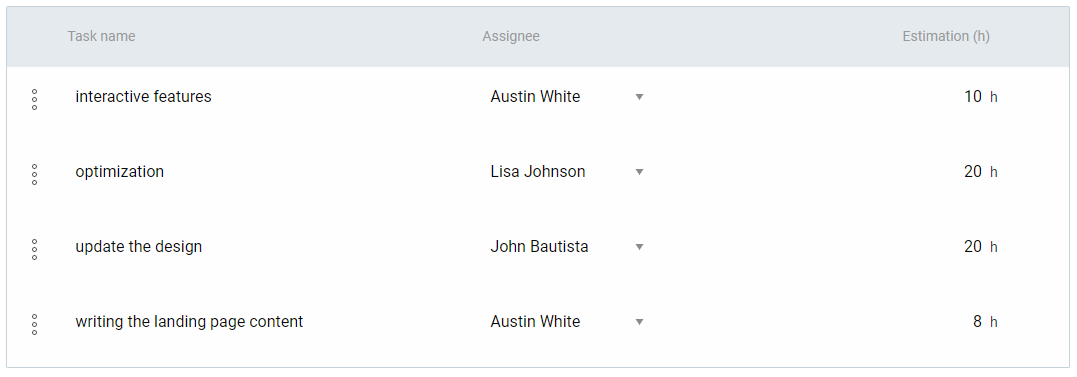A screen capture displaying a task management interface with a gray border at the top, featuring headers labeled "Task Name," "Assignee," and "Estimation (H)." Below, the tasks listed with bullet points include "Interactive Features," "Optimization," "Update the Design," and "Writing the Landing Page Content." Each task is assigned to an individual and includes an estimated completion time. The assignees are Austin White (Interactive Features, 10 hours), Lisa Johnson (Optimization, 20 hours), John Batista (Update the Design, 20 hours), and Austin White again (Writing the Landing Page Content, 8 hours). The interface is neatly organized with clear, black font and a thin gray border encapsulating the table. No additional elements or objects of note are present in this simple, easy-to-read layout.